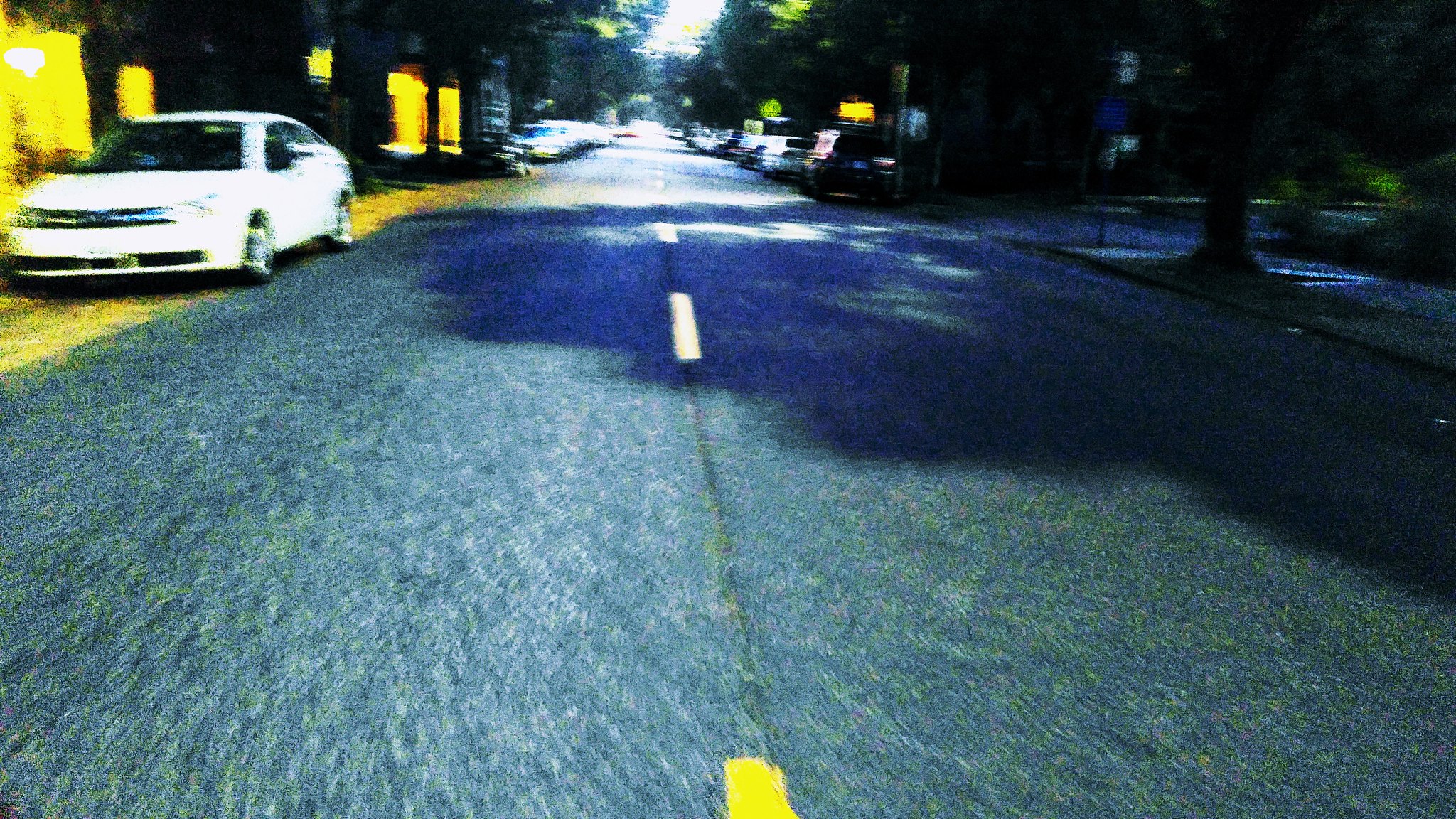This color photograph, taken outdoors during daytime, depicts a slightly skewed street scene from the perspective of a vehicle or person positioned on the road. The street features a white dashed line down its center, although the nearest dash is yellow, an anomaly likely due to exposure issues, which also give the road an unusual blend of white, gray, green, and yellow hues. On the left shoulder of the street, a white car is parked, aligned with a row of houses adorned with illuminated porch lights. Further along, more cars are parked in a line on both sides of the street, suggesting a heavily populated or urban area. The right side of the road features a tree near the sidewalk, along with additional trees and greenery lining the street, interspersed with small pedestrian signposts. Despite the photograph's blurred quality, the scene remains discernible with no visible people or text, emphasizing a calm, residential street environment.